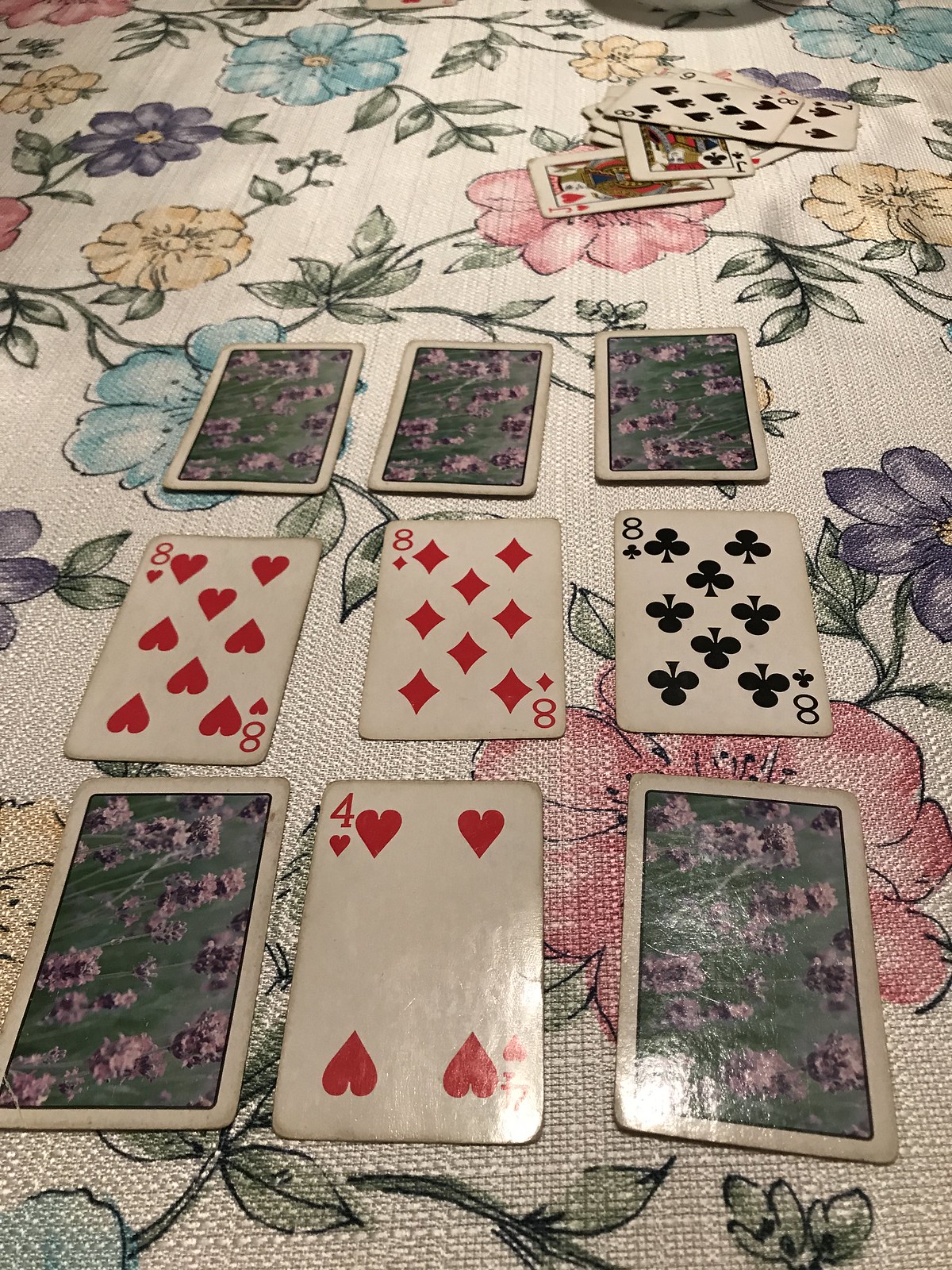In this image, a vibrant card game is unfolding atop a richly textured, off-white floral tablecloth. The tablecloth showcases an array of colorful flowers in shades of purple, yellow, blue, and pink, all interconnected by delicate green stems, with a clear display of the sewing texture especially noticeable towards the bottom of the photograph. In the top right-hand corner, there is a scattered pile of cards, prominently featuring the eight of spades and some jacks. Centrally, a neat 3x3 grid of nine cards is laid out. The top row consists of three cards, all face down. The second row reveals three face-up eights, vividly displayed. The bottom row includes a mix: a face-down card, the four of hearts, and another face-down card. The face-down cards are decorated with a lilac floral design against an off-white background, bordered with a black outline. Notably, there is a subtle reflection on a few cards, most prominently towards the bottom right-hand side of the image, adding an extra layer of detail and realism.